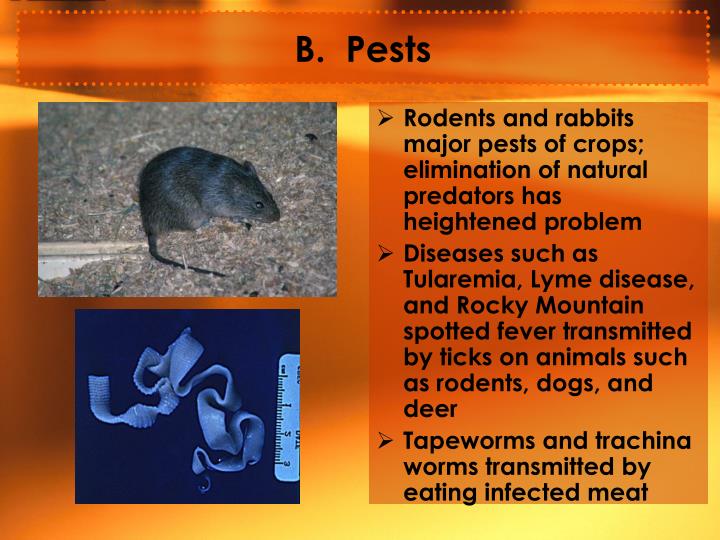The PowerPoint slide, titled "B. Pests" in black text on a red banner, features an orange and yellow gradient background. In the lower left section, there are two images: the first is a rectangular photo of a dark gray mouse on a light gray-brown background, and below it is a smaller square image with blue hues displaying a coiled, ribbon-like structure with ruler markings on it. On the right side, there is a block of black text with three bullet points. The first bullet states, "Rodents and rabbits are major pests of crops; the elimination of natural predators has heightened the problem." The second bullet point reads, "Diseases such as tularemia, Lyme disease, and Rocky Mountain spotted fever are transmitted by ticks on animals such as rodents, dogs, and deer." The third and final bullet mentions, "Tapeworms and trichina worms are transmitted by eating infected meat."